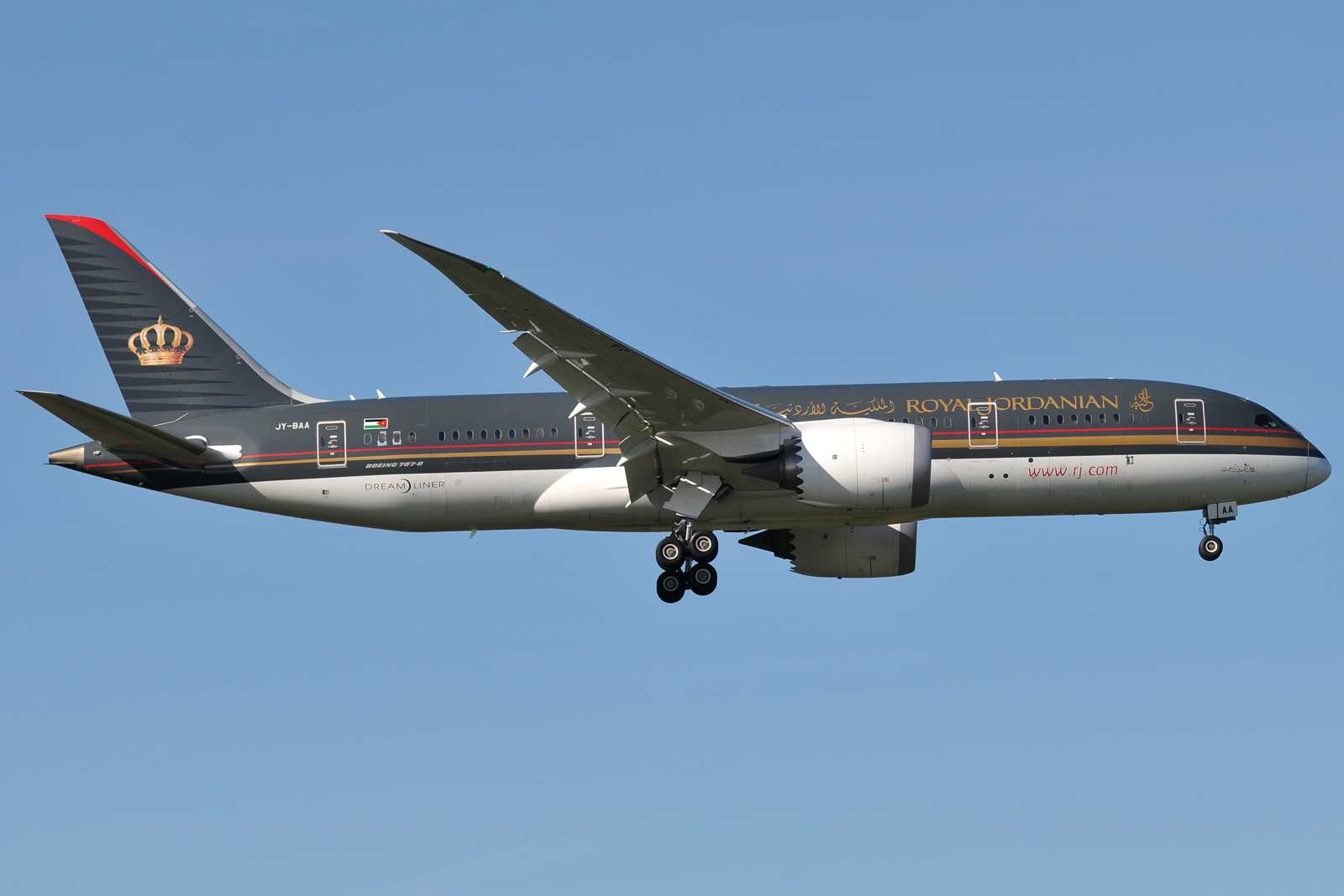This photograph captures a modern Royal Jordanian jet airplane soaring through a clear blue sky, its landing gear extended, indicating it is either taking off or preparing to land. The aircraft's sleek design features a distinct color scheme: the upper part of the fuselage is a striking black, transitioning to a pristine white on the lower half. A pair of bold stripes—a golden stripe and a red stripe—span the length of the aircraft along the black upper section. The sides of the plane prominently display the text "Royal Jordanian" in elegant golden lettering. The tail fin is adorned with a regal crown emblem, signaling the airline's royal heritage, and a national flag is situated next to the doors. Additionally, the airline's website, www.rj.com, can be seen on the plane. The image offers a slightly upward perspective, capturing the airplane in its entirety against the vast expanse of the blue sky, with ample space above and below to highlight its graceful presence.